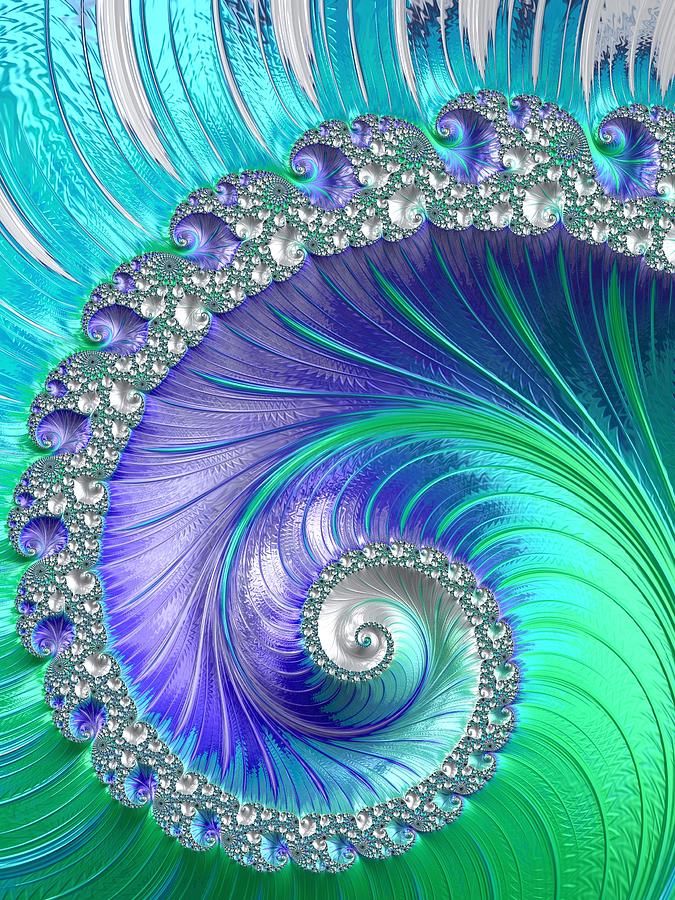This vertical abstract art piece features a central spiral design with an intricate array of smaller spirals nested within it. The artwork evokes the vibrant and iridescent beauty of a peacock, employing a rich palette that transitions from light to dark hues of green, turquoise, purple, violet, and blue. The spiral begins at the center with a white or silvery core and unfurls outward through turquoise, purple, and green gradients, culminating in a turquoise outline. 

The edges of the outermost spirals are meticulously encrusted with clear gemstones, adding a sparkling, textured detail reminiscent of embedded diamonds or cubic zirconias. Each sub-spiral echoes the larger one, contributing to a mesmerizing sense of depth and motion, creating an overall feel that is both feather-like and wave-like in its fluidity. This piece, digitally created, captures the hallucinogenic essence of a DMT experience, as suggested by its dreamlike, almost otherworldly color transitions and intricate details. In the very center of the lowest part of the spiral, a singular blue dot stands out, drawing the viewer’s eye and adding an intriguing focal point to the piece.